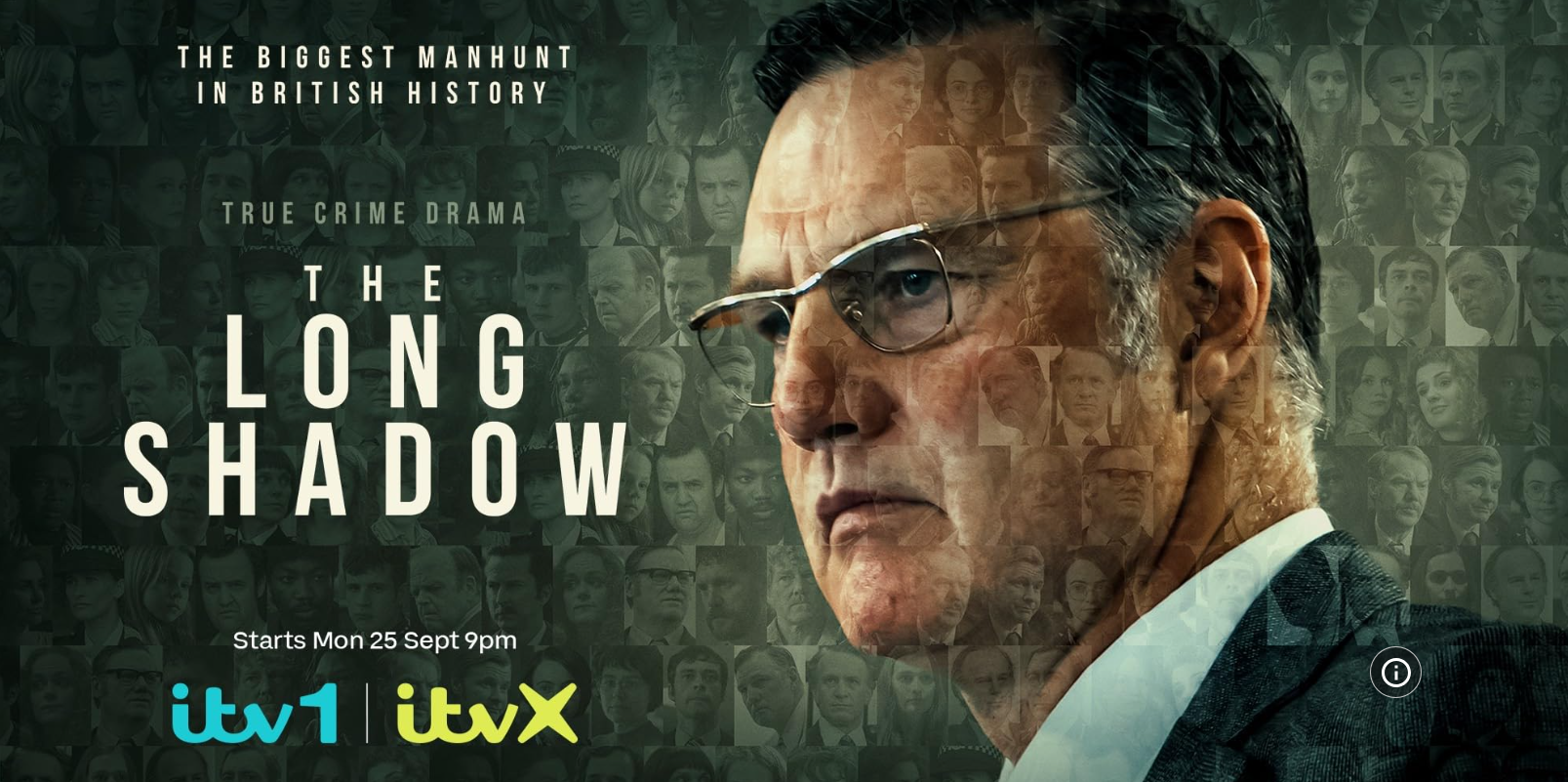The image is a promotional advertisement for a TV series, characterized by a horizontally aligned, landscape orientation. The composition is divided into two main sections. On the left side, in white uppercase letters at the top, the text reads "THE BIGGEST MANHUNT," followed by the centered phrase "IN BRITISH HISTORY." Below this, in light gray uppercase letters, the words "TRUE CRIME DRAMA" are also centered. Dominating the center of this section, the title "THE LONG SHADOW" is displayed in the largest text, arranged with "THE" slightly smaller but still in uppercase. Further down, in mixed uppercase and lowercase letters, it says "Starts Monday 25th September 9pm." Beneath that, in medium-sized blue cursive text, "itv1" is printed, followed by a vertical dividing line, with "itvx" in yellow cursive text alongside it.

The right side of the image features a man who appears to be in his early 50s, a Caucasian with salt-and-pepper hair and wire-rimmed glasses, wearing a black blazer over a white shirt. He has a serious, contemplative expression, looking off to the viewer's left. The background behind him consists of a mosaic or collage of numerous blurred faces, both male and female, rendered in a greenish hue. This pattern subtly extends over the man's face, creating a layered effect. In the upper left area of his collar, a white 'i' inside a white circle, suggests an interactive element for more information, indicating this might be a modern digital screenshot. The overall style of the design combines photographic realism with special photo filters, graphic elements, and typography.